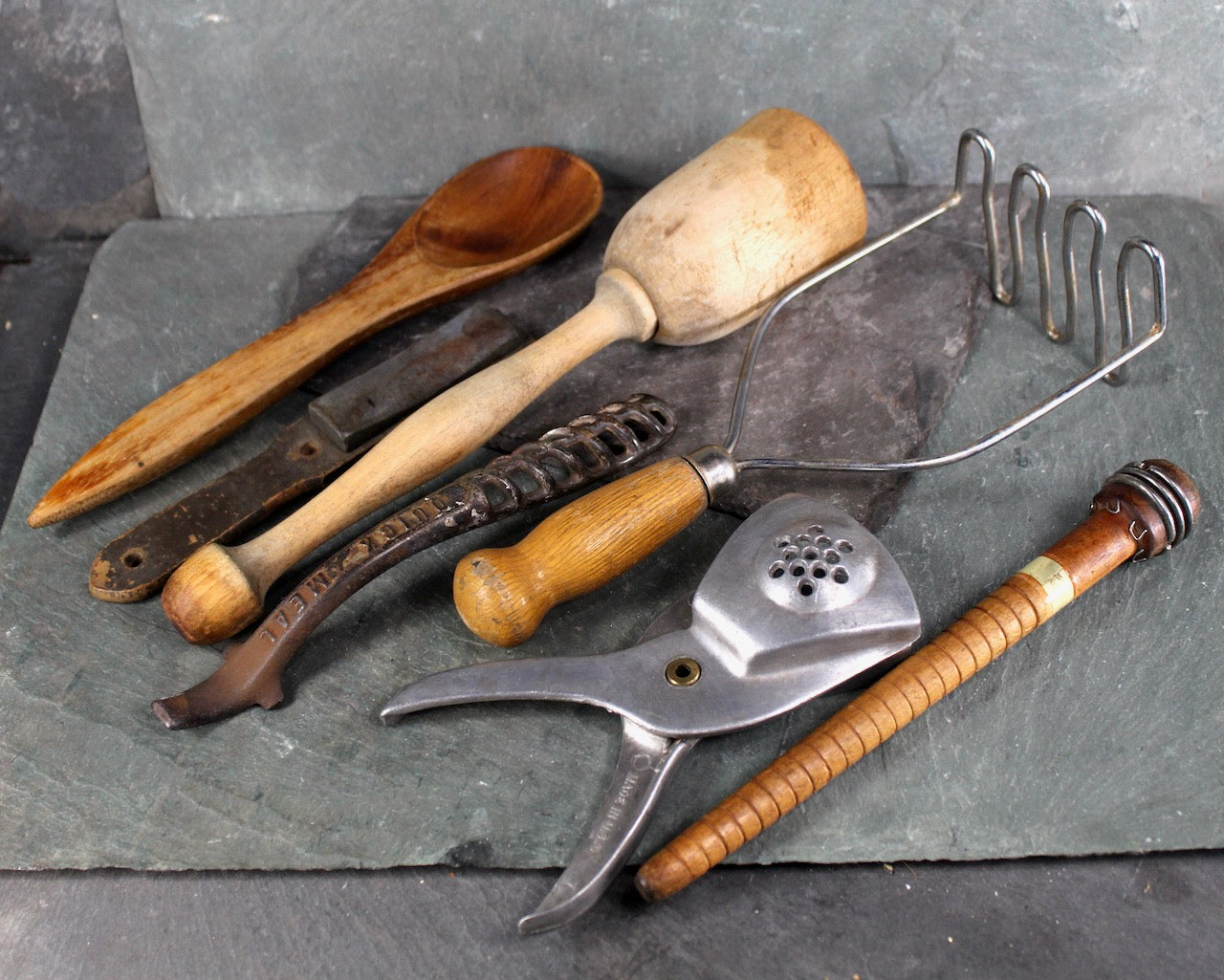This horizontal rectangular image showcases a collection of vintage kitchen utensils, most of which have been replaced by modern equipment. These worn tools, primarily made of wood and metal, are laid out on what appears to be a sheet of iron or possibly a stone shelf with a green mat. The well-used wooden spoon, dark from years of handling and use, is positioned in the upper left corner, leaning against the wall. Next to it is another mysterious wooden object, possibly for pounding meat. At the center, there's a sizable wooden tool that resembles a hammer. Other notable implements include an old-fashioned wire potato masher, a metal juicer, and several other metal tools whose exact purposes are uncertain. One such object, resembling a wrench, is visible, while another tool with a long pole and a cup-like end is situated towards the right. All together, there are seven distinct, timeworn kitchen tools, each telling a story of a bygone era of culinary arts.